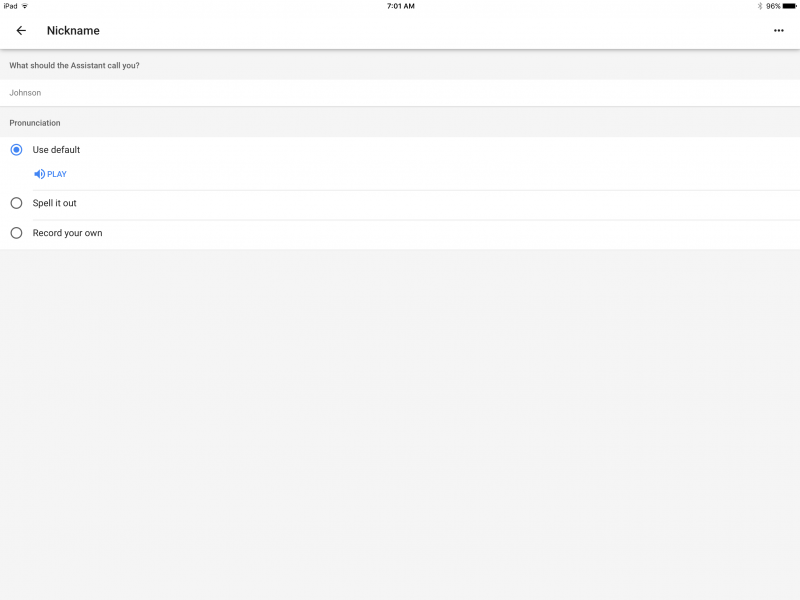The image showcases the screen of an iPad device. At the top left corner, the label "iPad" confirms the device type, while the center of the status bar indicates a strong signal. The time displayed is 7:01 a.m., and the battery life is at 96%. Just below the status bar, the screen focuses on the "Nickname" settings for a digital assistant.

In the initial grey panel, the text prompts the user with the question, "What should the assistant call you?" The currently set nickname is "Johnson." Directly beneath this, another grey panel is dedicated to pronunciation options. The default setting is employed, with a blue play button available for playback testing. Besides the default option, users have the choice to "Spell it out" or "Record your own" audio sample for pronunciation customization.

The lower two-thirds of the screen is occupied by a large grey panel, devoid of any visible content, maintaining a uniform grey appearance without additional details or features.